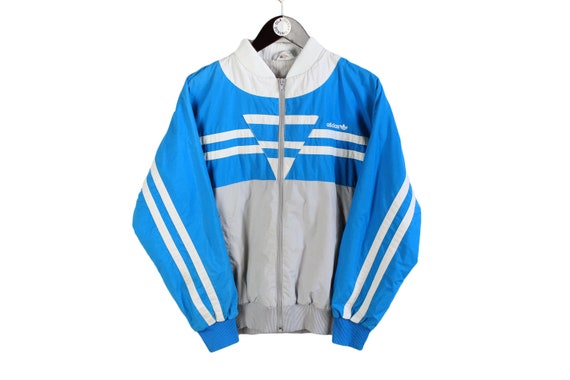The image is a detailed photograph of an athletic jacket, likely used for advertisement purposes, presented against a clean white background. The jacket is displayed on a hanger, which is predominantly dark wood with a distinct white circle at its center.

The jacket itself features a striking design with a variety of colors and intricate details. It boasts a high, white collar that complements the blue fabric dominating the upper portion, including the sleeves and chest area. A pair of white stripes runs horizontally from sleeve to sleeve, intersected by an inverted triangle at the center chest, creating a visually appealing pattern.

This jacket, zipped fully up in the middle with a gray zipper, transitions below the chest into a lighter gray fabric, which appears ruched or ruffled, suggesting an elasticated waistband. The cuffs of the sleeves also have a similar gathered design, indicating a snugger fit at the wrists. Upon closer inspection, the jacket showcases an Adidas emblem in white, located on the upper chest area, reinforcing the athletic theme. There’s also a tag visible at the back, adding to the authenticity and detail of the image.